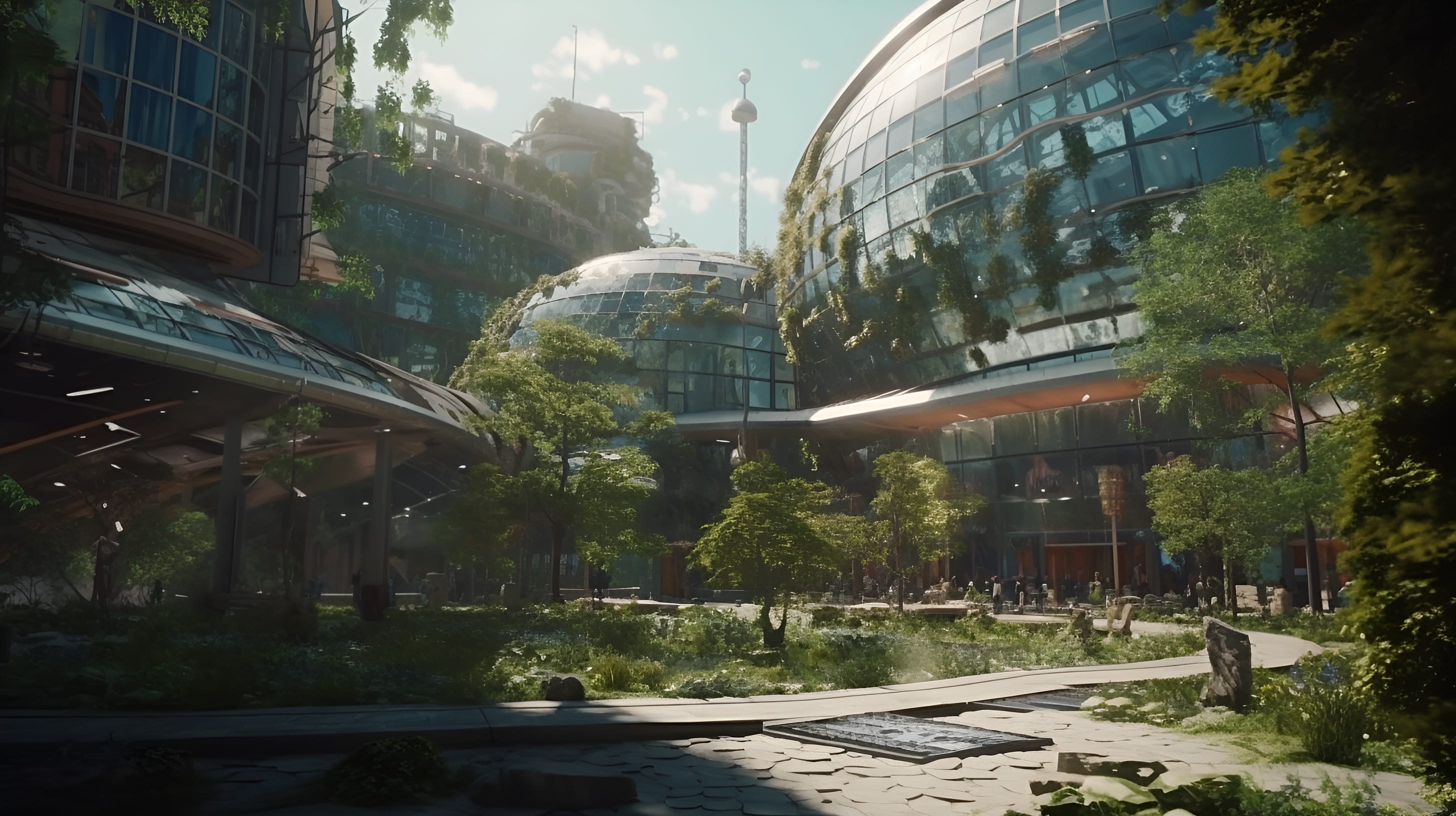The image depicts a futuristic, utopian setting characterized by a lush garden courtyard enclosed by several round, dome-like buildings made primarily of glass. These gleaming structures, resembling giant bubbles, feature roof designs that mimic planetary rings and are adorned with hanging greenery. The central garden is vibrant with trees and various plants, while stone pathways crisscross the area, connecting the buildings. The scene is bathed in sunlight, with a clear blue sky overhead. The combination of advanced architectural design and abundant plant life suggests a harmonious blend of technology and nature.